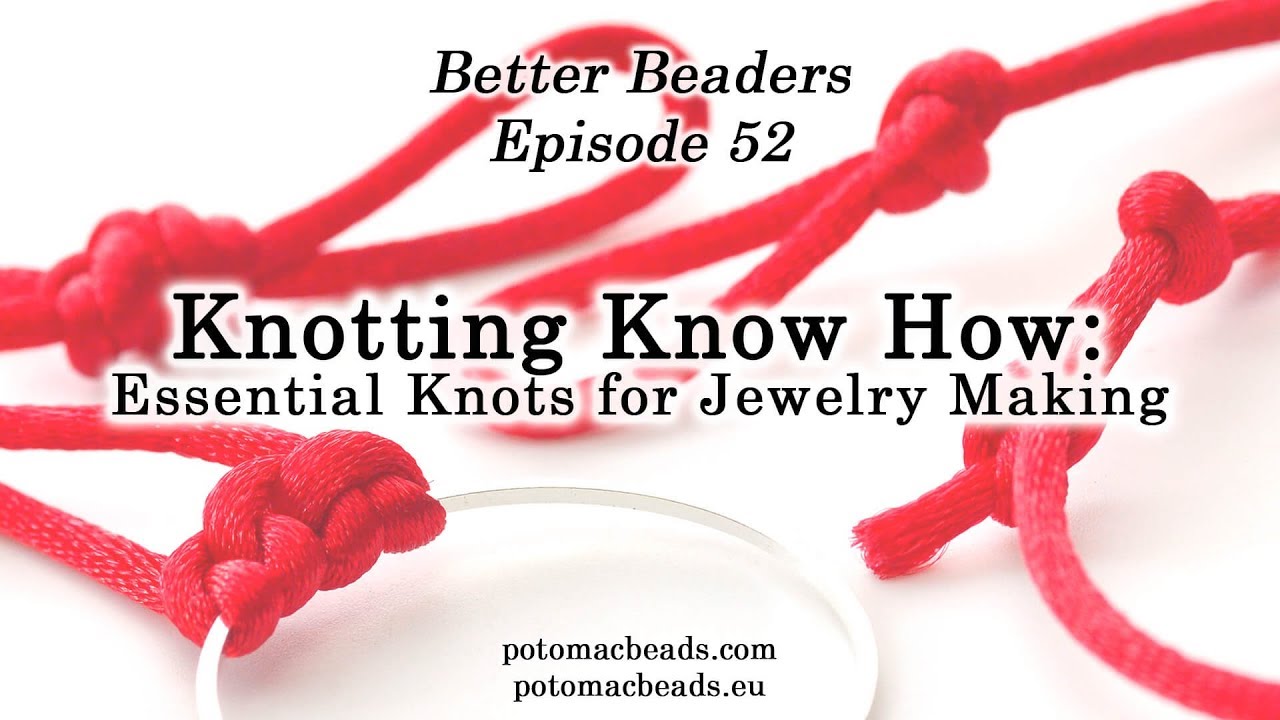The image is a detailed color photograph in landscape orientation, featuring vivid red cords tied into several intricate knots, which are essential for jewelry making. The background is a soft pale pink, and the photograph captures a silver loop at the bottom left corner, partially cropped and casting a shadow, with a double-knotted red cord grasping it. At the top of the image, in capitalized black text, it reads "BETTER BEADERS EPISODE 52." Centered in the middle of the photo is a prominent black text with a white drop shadow that says "Knotting Know-How: Essential Knots for Jewelry Making." The bottom of the image displays two website URLs, PotomacBeads.com and PotomacBeads.eu, positioned inside the silver loop. The composition blends photographic realism with graphic design typography, clearly serving as an informative and visually appealing guide for better beadwork.